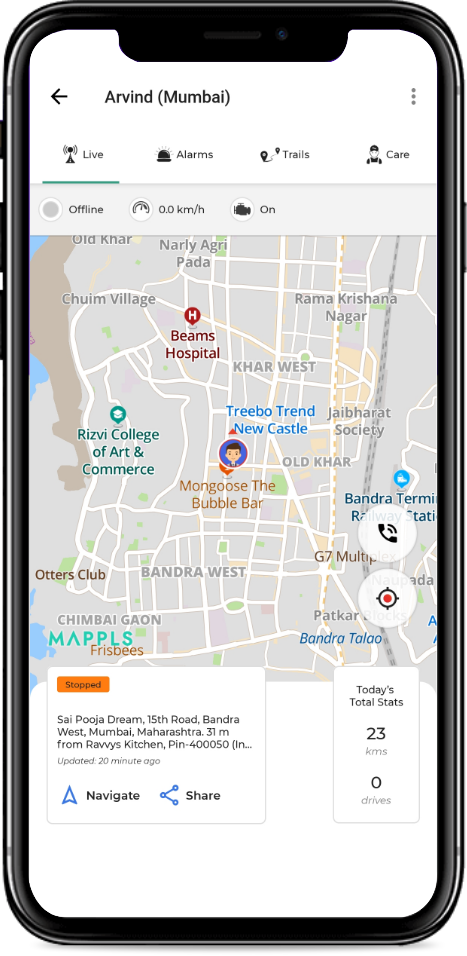The image depicts a digital rendering of a smartphone displaying a detailed screenshot in portrait mode. The exterior of the phone has a sleek design with a silver-to-black gradient and multiple buttons: two short and one long on the left side, and one long on the right side.

Within the screenshot, a navigation interface is presented. At the top, there is a back arrow icon, followed by the text "ARVIND (Mumbai)" with the word "live" underlined in green. Below this, there are tabs labeled "live," "alarms," "trails," and "care."

The central part of the screenshot features a detailed map highlighting various locations, including Beams Hospital, Tribo Trend, Newcastle Mongoose, The Bubble Bar, and Ritz V College of Art and Commerce.

Under the map, there are four white information cards. The left card, marked with an orange "stopped" label, details a location: "Pooja Dream, 15th Road, Bandra West, Mumbai, Maharashtra," situated 31 miles from "Ravi's Kitchen." Options to "navigate there" or "share" are provided.

The right card displays "today's total stats" which show "23" and "zero drives," suggesting the app might be tracking driving statistics or related information.